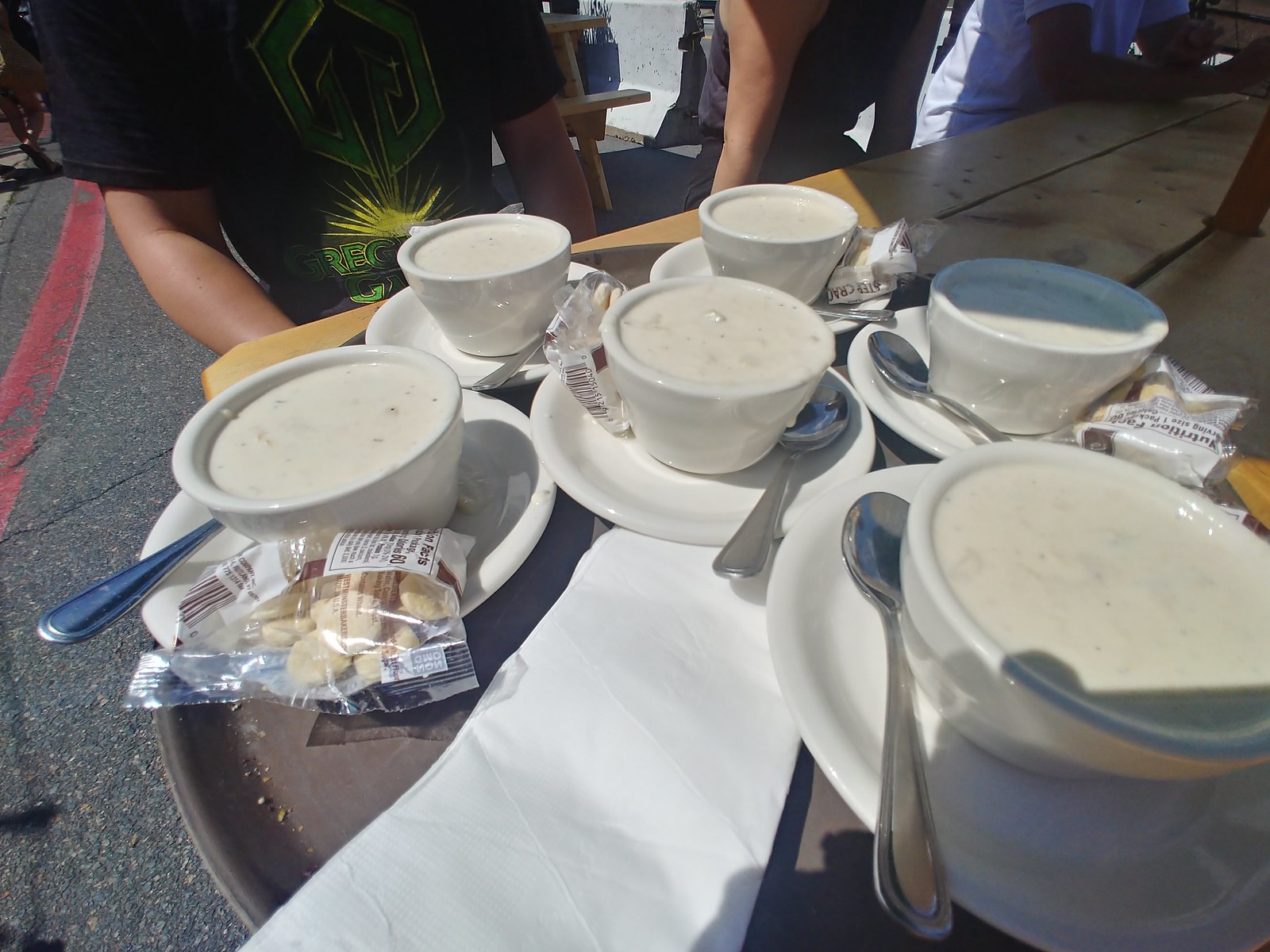The photograph depicts an outdoor dining setting on a pavement with a faint red-painted stripe and visible sunlight. The focal point is a wooden picnic table with a central hole for an umbrella pole. At the end of the table, a waiter in a black shirt with a green logo, showcasing tan arms, holds a round tray. The tray carries six white bowls of creamy New England clam chowder, each placed on a small plate accompanied by a soup spoon and packets of oyster crackers. Around the table, four people are seated, wearing different colors: black, purple, and blue shirts. Additional picnic tables and benches can be seen in the background, adding to the casual, outdoor ambiance of the setting.